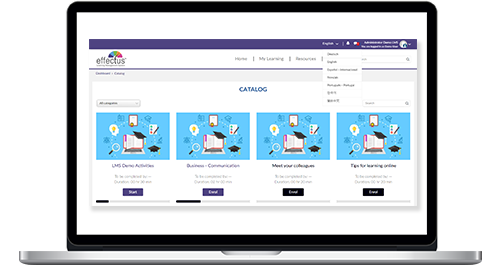The image showcases a silver laptop positioned head-on against a white background. The laptop's front edge and shell are silver, while the bezel surrounding the screen is black. The laptop screen displays a website with a white background, featuring a dark blue banner at the top. Just below the banner, there is a logo depicting an arched rainbow with black text underneath that appears to read "Effectus." Towards the top of the screen, there are navigation options that include "Home," "My Learning," and an unreadable third option. Below this navigation bar, the word "Catalog" is prominently displayed in bright blue, leading to a drop-down menu. The main section of the screen showcases four rectangular images with a blue background, each depicting a book surrounded by orbiting icons. The text beneath each image varies, with the first one labeled "LMS" and the second possibly reading "Business Communication." The texts under the third and fourth images are unreadable. Each image has a button positioned beneath it.